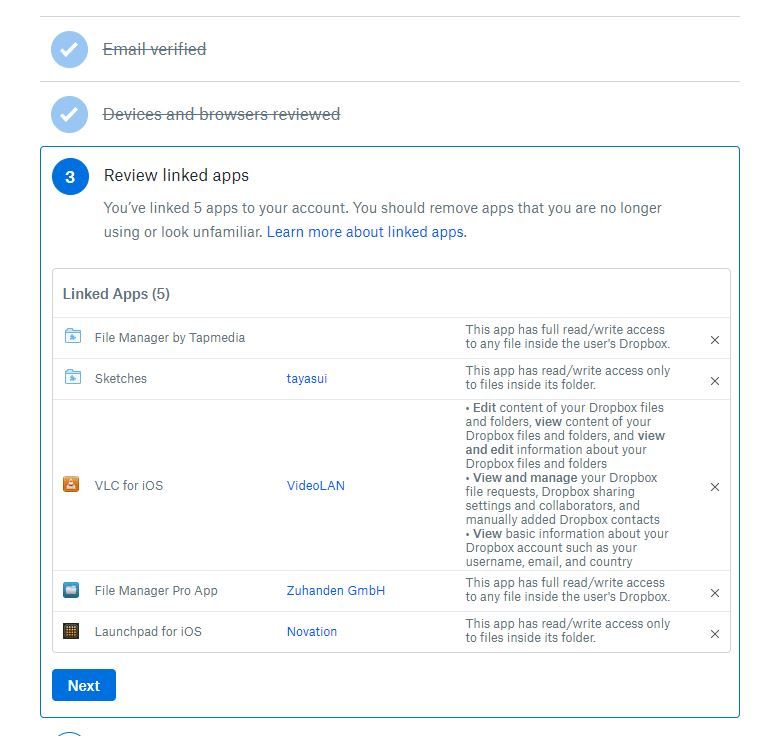### Detailed Image Caption

The image presented is a vertically structured interface, approximately 20% taller than it is wide, with a white background.

- **Top Section**:
  - A thin gray horizontal bar serves as a divider.
  - Below the bar, there is a blue circle containing a white checkmark, signifying completion.
  - To the right of the circle, the text "Email Verified" appears, struck through with a horizontal line, indicating the task is already completed.

- **Middle Section**:
  - Another gray horizontal line separates this section from the above.
  - Again, a blue circle with a white checkmark is present on the left.
  - To the right, the text "Devices and Browsers Reviewed" is displayed, also struck through to denote completion.

- **Main Content Area**:
  - A green square outlines the remaining content, providing a distinct border.
  - Inside the green square, at the top-left corner, a blue circle with the number "3" can be seen, signifying the third step or item.
  - Adjacent to the blue circle, black text reads "Review Linked Apps."

- **Instructional Text**:
  - Below the "Review Linked Apps" heading, a message in black text states: "You've linked five apps to your account. You should remove apps that you are no longer using or look unfamiliar."
  - To the right of this message, a blue hyperlink reads: "Learn more about linked apps."

- **List of Linked Apps**:
  - The section titled "Linked Apps" lists five applications linked to the account:
    1. File Manager by Tap Media
    2. Sketches
    3. VLC for iOS
    4. File Manager Pro App
    5. Launchpad for iOS

Each part of the image offers clear, distinct instructions and information about managing linked applications for an account.